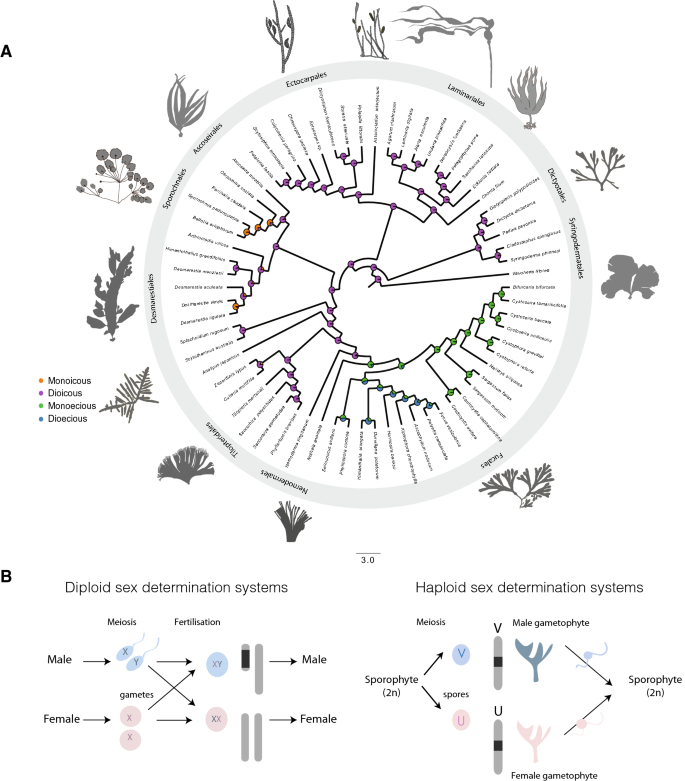The illustration, likely from a biology textbook, presents a detailed explanation of biological processes related to plant types and sex determination systems. The top part, labeled as Figure A, features a central circular diagram with a light gray outline. Inside this wheel, the Italian names for various plant materials are inscribed in inward-facing black italic text. Interconnecting spokes, denoted by long black lines and dotted with orange and green circles at intersections, extend from the center. Surrounding the outer edge of the wheel are light and dark gray depictions of different shrubbery and plant shapes. To the left, a color-coded key uses orange, purple, green, and blue dots to label terms like Monoecious, Dioecious, Monoecious, and Dioecious.

Below this, labeled Figure B, are two columns detailing sex determination systems. The left column, titled "Diploid Sex Determination Systems," illustrates a sequence starting with meiosis and fertilization. It includes color-coded blue sperm (labeled with X and Y) and light pink eggs (labeled XX), with arrows indicating the resulting male (XY) and female (XX) chromosomes. The right column explains "Haploid Sex Determination Systems" starting with a sporophyte denoted as 2n. The diagram shows a division into V (blue) and U (orangey pink), with labels for spores and vertical pill-like structures. It continues with graphical representations of tree-like structures in green (male gametophyte) and pink (female gametophyte), concluding with another sporophyte labeled 2n. The comprehensive depiction uses shades of gray, black, blue, and pink to convey complex biological systems and plant classifications.